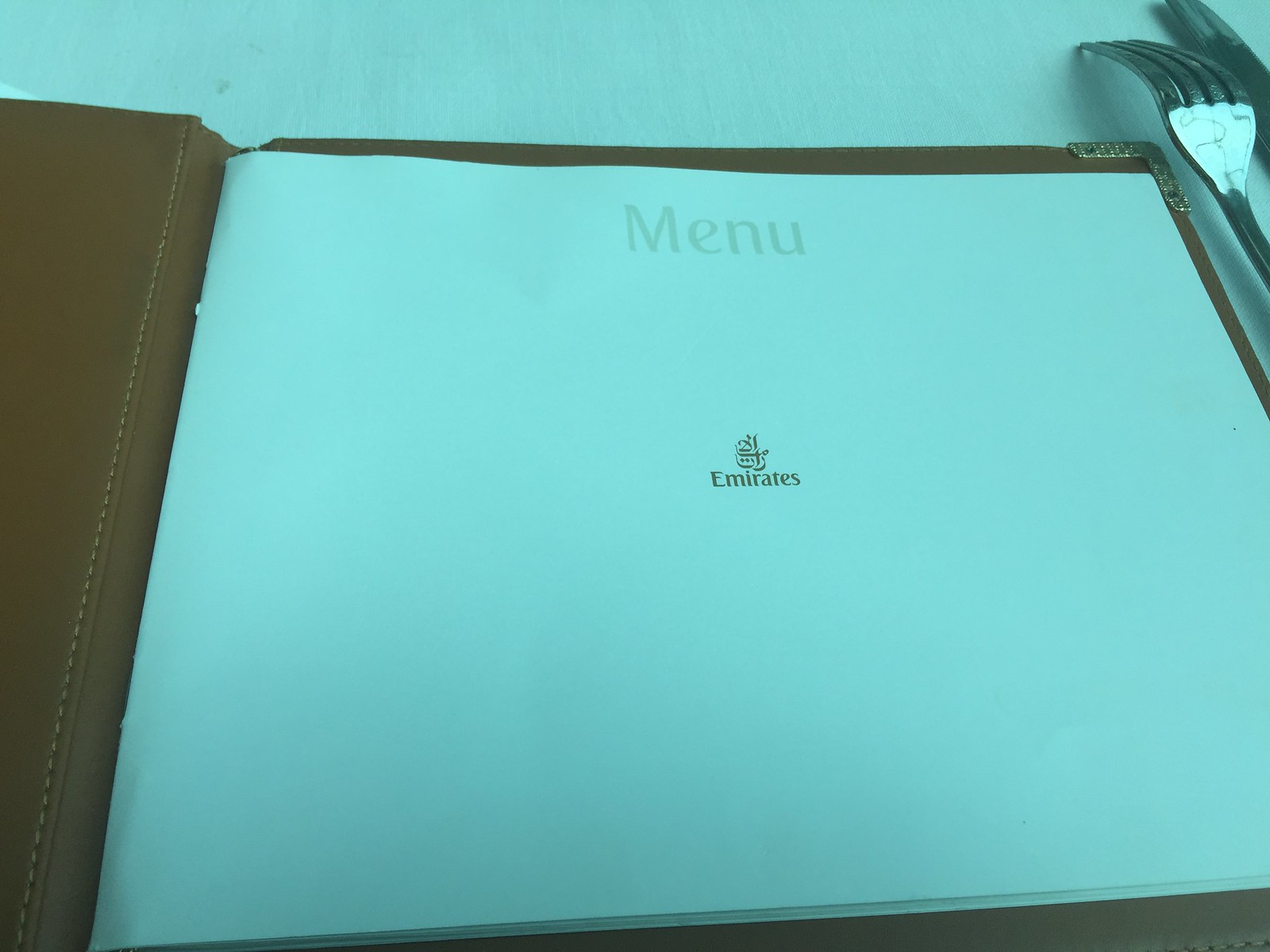A top-down image showcases an elegant airline menu setup. The scene captures a pristine white tablecloth with the edge visible at the top of the frame. On the right side, a fork lies prongs down next to a butter knife, placed neatly. The focal point is a simple, sophisticated menu—a white piece of paper adorned with gold lettering. At the top of the menu, "Emirates" is inscribed in light text, complemented by a small sword logo in the center. Behind the menu, the background features a luxurious brown leather panel with distinct gold stitching, also bearing the "Emirates" logo. The menu's design is minimalistic, with a gold triangle accent at the top right corner. The overall composition exudes a sense of luxury and refinement typical of an Emirates airliner.